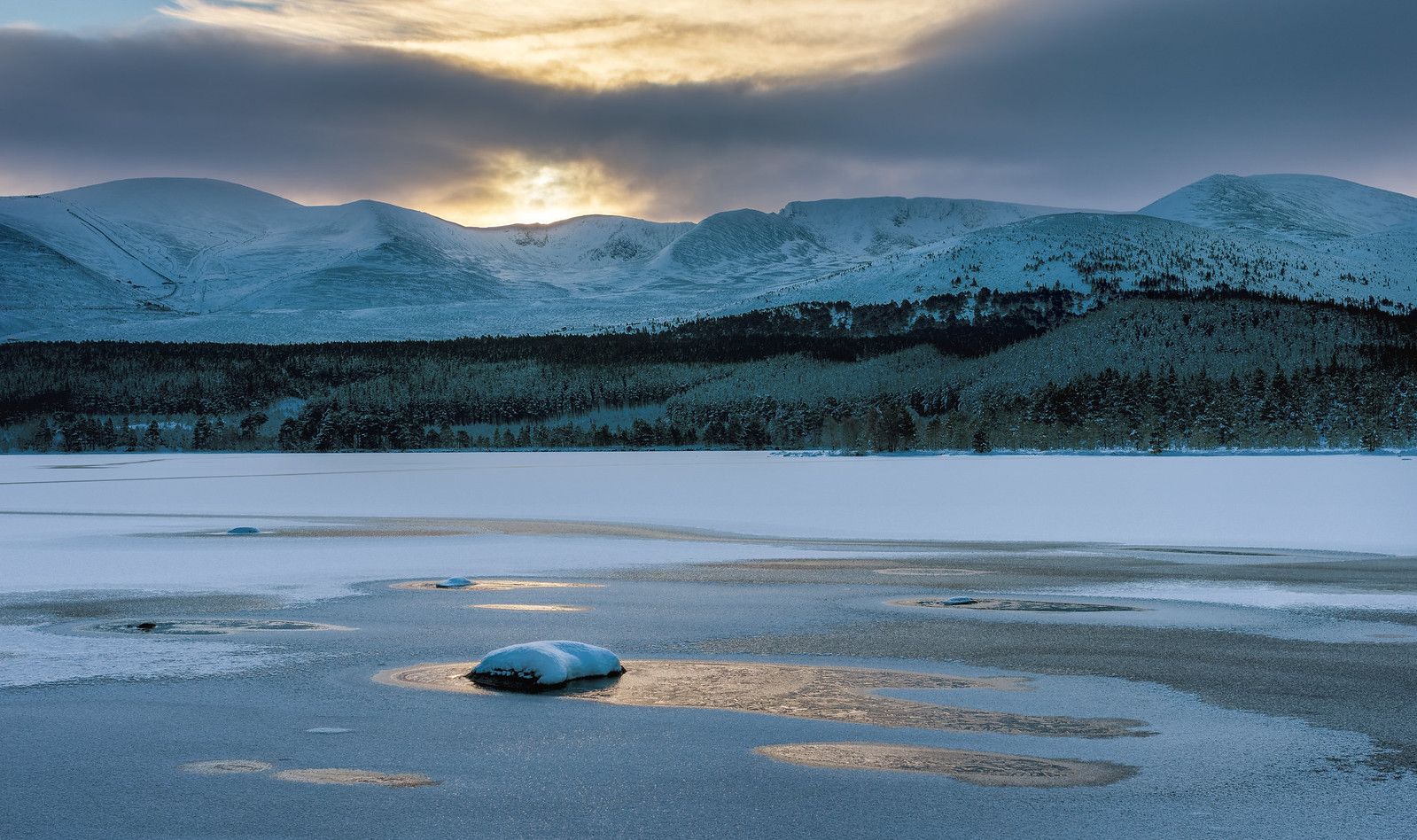The photograph captures a serene yet ominous winter scene in a mountainous area featuring a partially frozen lake. The lake is predominantly iced over, with patches of water and thin, unstable ice that looks as if it might be starting to melt. Snow covers parts of the ice and obscures other sections, creating a reflective surface in some areas. A boulder juts out noticeably from the ice halfway across the lake, accompanied by other smaller rocks protruding from the water. The shoreline, entirely enveloped in snow, leads to a dense forest of snow-covered evergreen trees that extend up to a range of snow-clad mountains in the background. The sky is heavily overcast and gray, casting a wintry and stormy ambiance over the landscape. A hint of sunlight attempts to break through the clouds, suggesting the possibility of a sunrise or sunset, as faint yellow hues reflect off the lake's surface. Additionally, an indistinct snow-covered object, resembling a pillow, lies on the ice, adding a curious element to the wintry tableau.